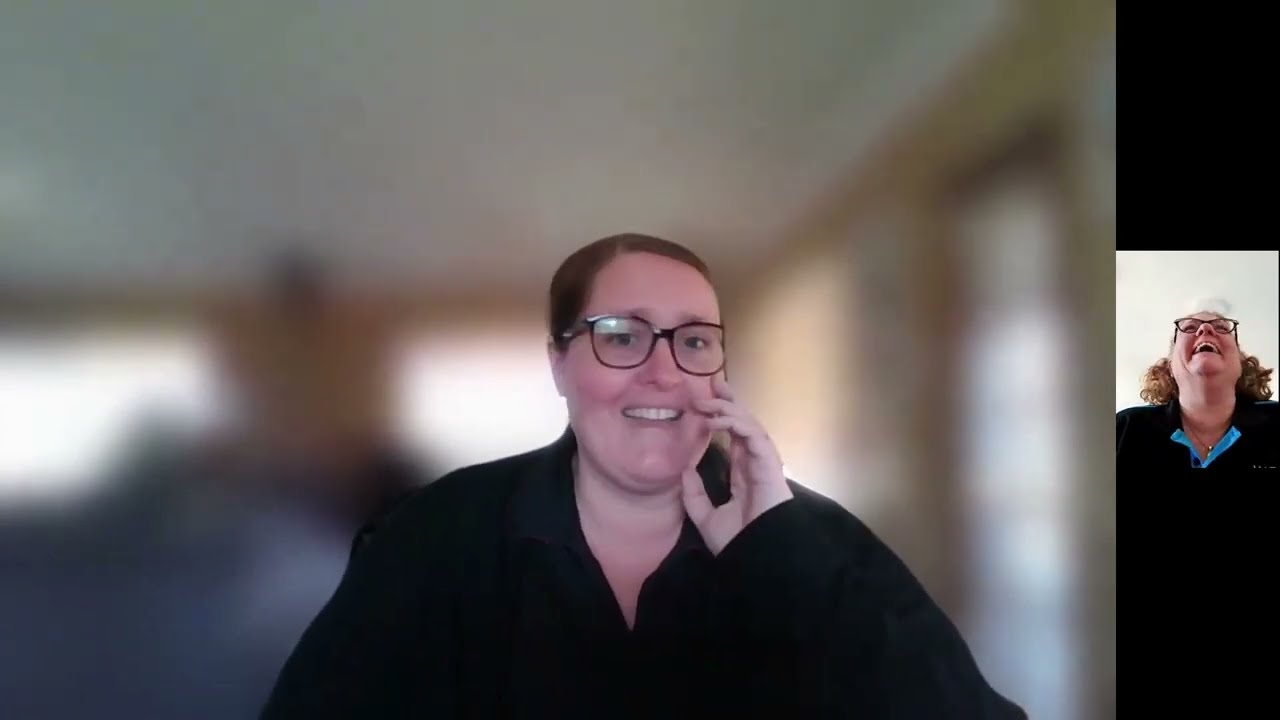The image is a screen grab from a live video conference featuring two women. The woman occupying most of the screen appears to be in her 30s, with her hair swept back, possibly in a bun, and she is wearing glasses with dark frames. She is dressed in a long-sleeve black blouse, and her background is heavily blurred, suggesting an indoor setting with several windows and a door slightly visible. She is smiling with her left hand touching her face, engaged in a lively discussion. On the right-hand side, there is a smaller image of another woman, likely middle-aged with shoulder-length light sandy blonde or brown hair and wearing glasses. She is dressed in a black blouse with a blue or turquoise collar and a necklace. Her head is thrown back, and her mouth is open, laughing hysterically at something the main woman has said. The scene depicts a cheerful and engaging interaction between the two women during their video call.